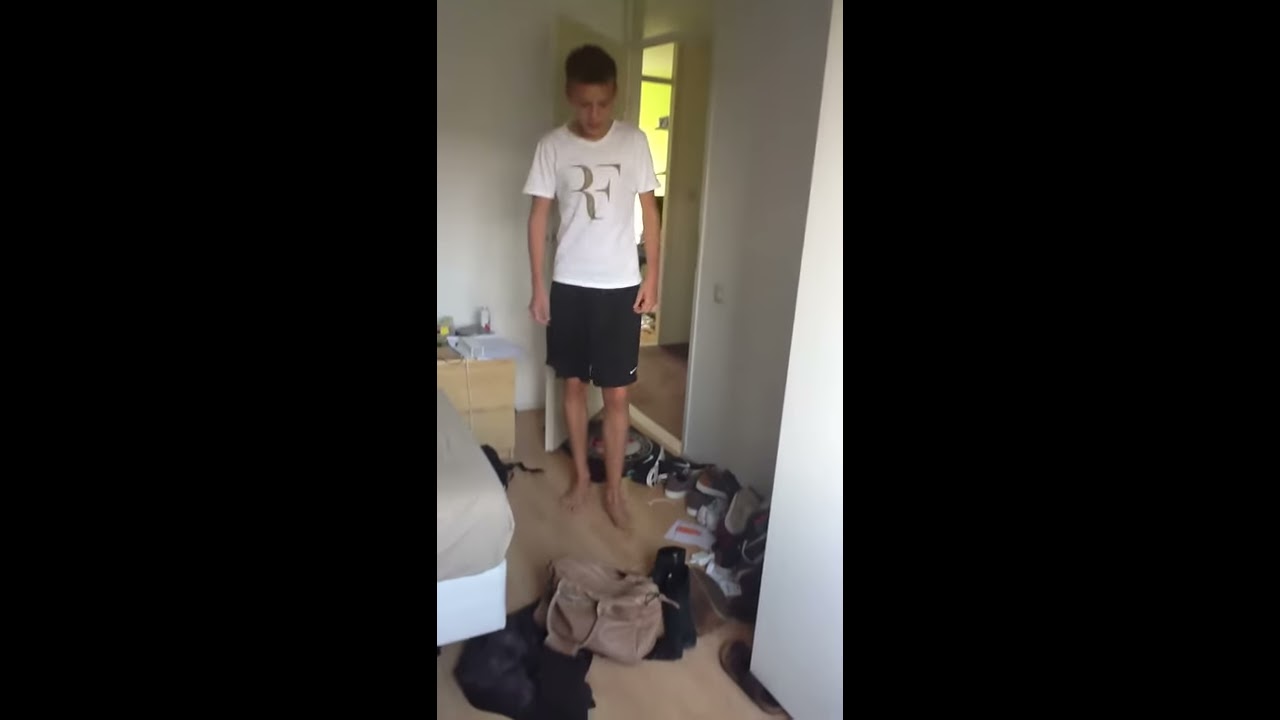The image depicts a young boy standing barefoot in a bedroom on a light brown carpet, looking down at a light brown leather bag in front of him. He is wearing a white t-shirt with faint outlines of the letters "R" and "F" and black shorts featuring a white Nike logo on the end leg. His short brown hair frames his solemn expression. Surrounding his feet are numerous pairs of shoes scattered haphazardly across the floor. To his left, there is a bed and a bedside drawer, and behind him, an open doorway reveals a corridor. The walls are painted white, and the room is well-illuminated, with light from the corridor casting a glow through the doorway.